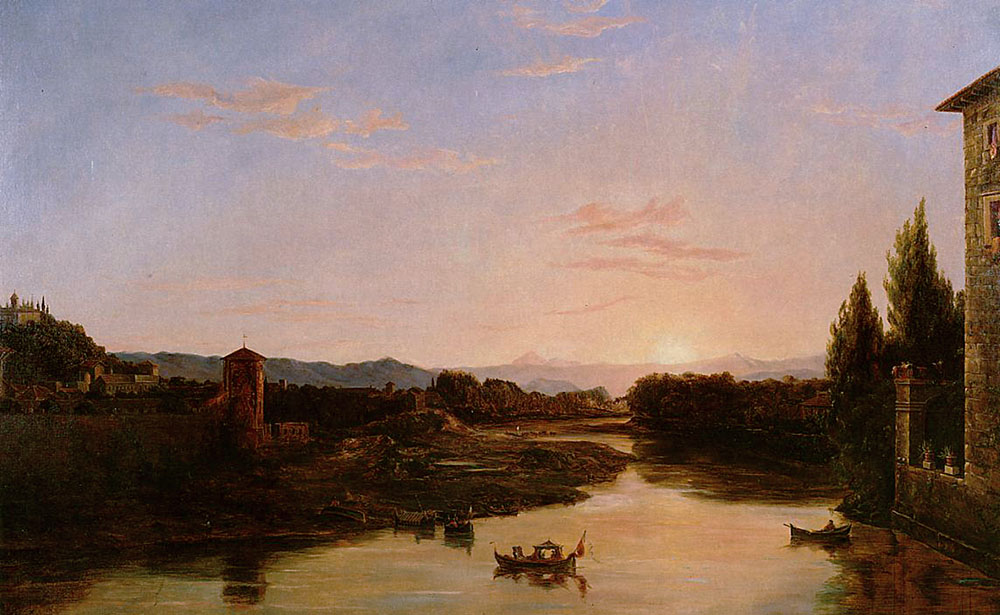The image is a horizontally aligned rectangular piece of artwork, likely a painting, depicting an outdoor scene under a vast, textured sky. The top half of the painting is dominated by the sky, painted mostly in shades of blue with occasional feathery clouds tinged in light gray and pink. Toward the middle, the bright white Sun is noticeable, positioned just above the horizon. 

Below the sky, the scene transitions to a landscape featuring a body of water that widens towards the foreground. Several small boats are scattered across the water, including one near the right bank, one in the middle, and two near the left bank. The water itself seems to reflect the sky with hues of pink and blue.

On the left side, the ground inclines up to a hill crowned with a building with steeples, surrounded by numerous trees. A brown tower is also visible lower on the hill. On the right side of the painting, there are tall trees in the foreground and a partially visible brown stone building that appears to include a tall tower. The entire scene is set against a backdrop of a mountain range visible on the horizon. The various colors used in the painting include blues, pinks, oranges, browns, tans, greens, light blues, grays, and blacks. The overall composition appears scattered yet harmonious, capturing the tranquil essence of an outdoor setting in the middle of the day.